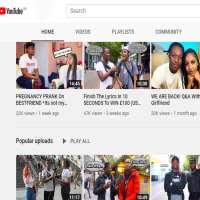Blurry and heavily cropped, this YouTube home page image starts from the top left where the familiar YouTube logo—a red bubble with a white play button at its center—and the word "YouTube" in bold black letters can be seen. To the right of the logo, a search bar with "search" written inside is visible. Below this, the screen has a white background with four tabs: Home, Videos, Playlists, and Community.

The image also shows three video thumbnails beneath these tabs. The first thumbnail features a man and a woman in conversation, the second displays two men seemingly engaged in a street interview, and the third depicts a couple facing the camera.

At the bottom row, there is a section labeled "Popular Uploads" with a "Play All" button adjacent to it. This section includes three video thumbnails, each showing people outside conducting street interviews.